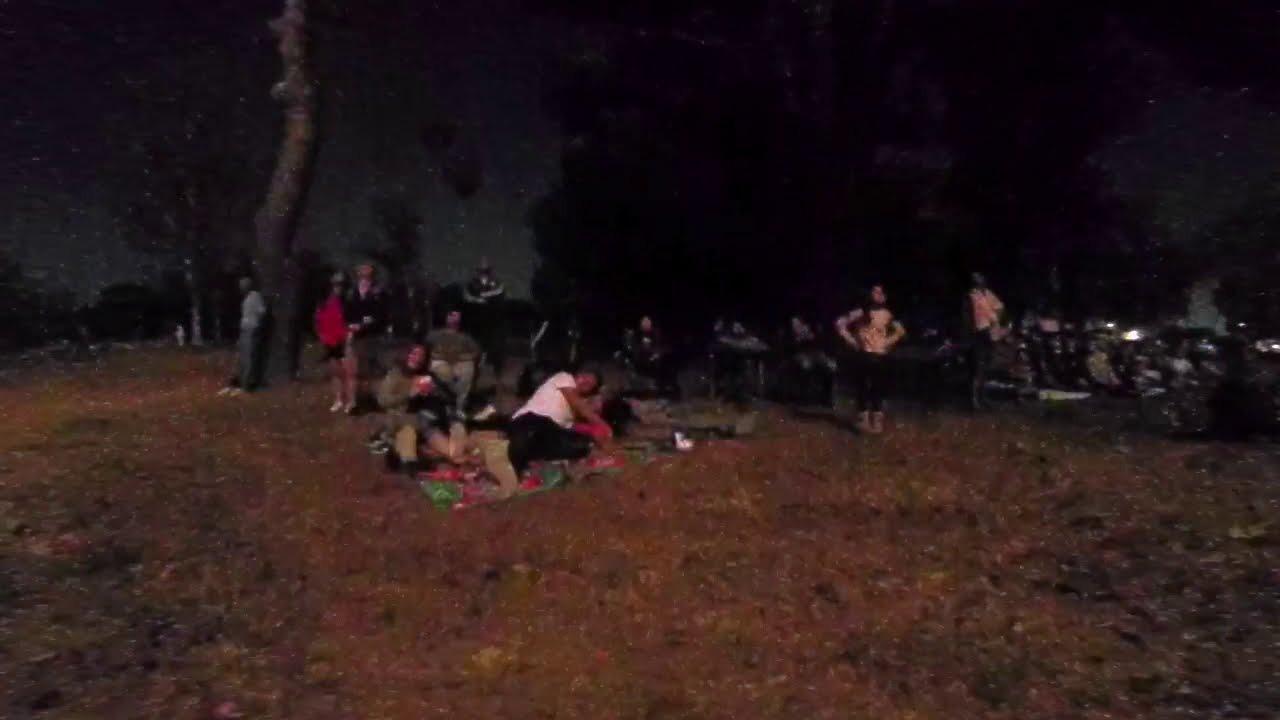In this grainy nighttime image, we see a group gathered in a field, potentially for a stargazing event, meteor shower, or fireworks display. The scene is dark, with minimal lighting provided by an orange glow, possibly from a bonfire just out of the camera's view. The central focus is on a picnic blanket in red and green hues, where several people are lying down. A man in black pants and a white t-shirt is prominent among them. There are about 13 to 20 people in total, spread across the field; some sit in lawn chairs, while others lean against a leafless tree, hinting that it might be autumn. The background hosts a row of motorcycles and the silhouettes of dark trees, emphasizing the clear night sky dotted with stars. The ground is a mix of brown and green, indicating a possibly worn field.